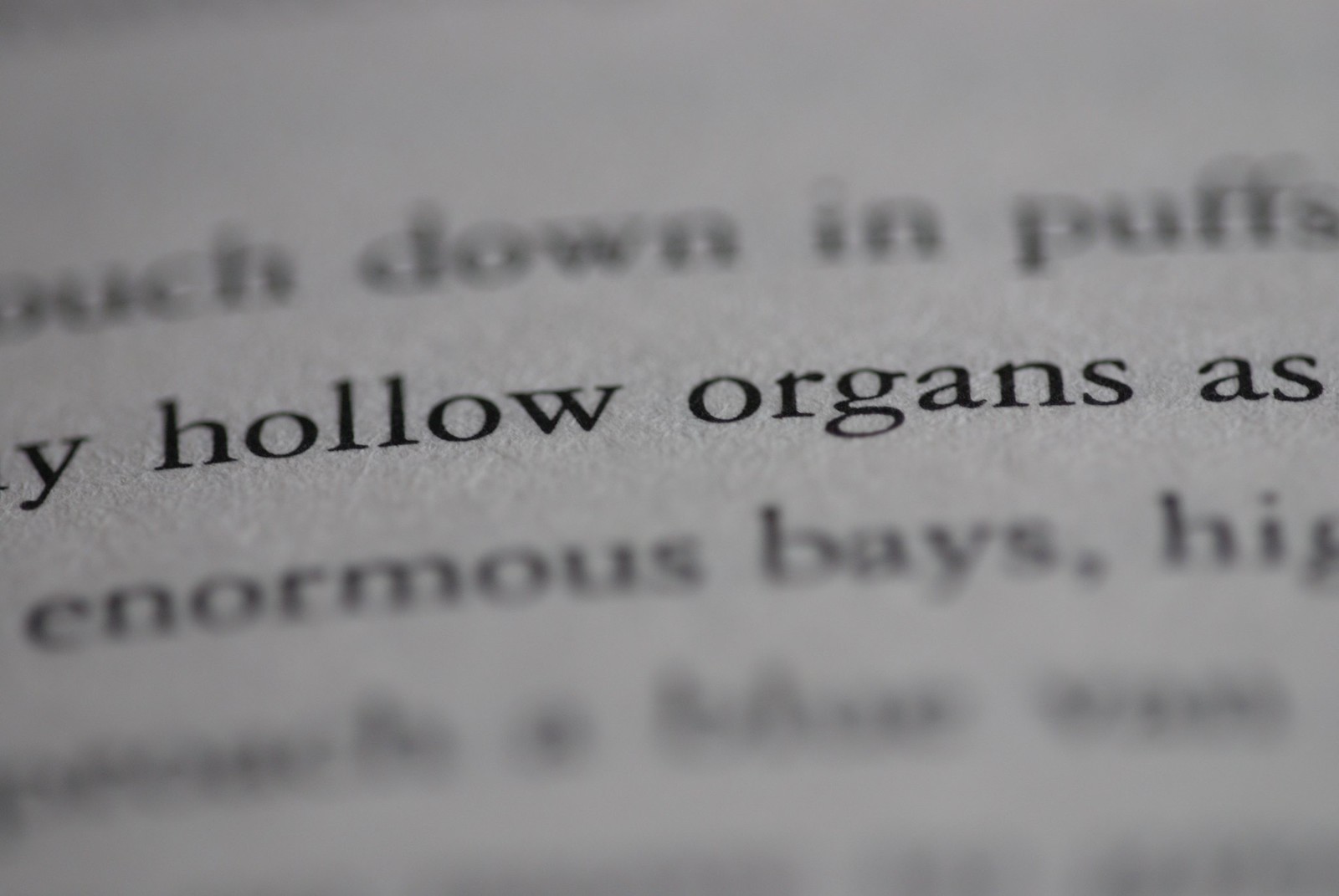The image is a horizontally aligned rectangular close-up of a book page with a gray, blurry background and no border. Across the center of the image is raised, clear text in dark black font reading "hollow organs as." Above this line, there is an unfocused and blurry line, barely legible, that seems to say, "much down in PUFFS." Following the clear "hollow organs as" line, the third line, also partially obscured and fuzzy, appears to read "enormous bays HI." The fourth and final line at the bottom of the image is unreadable due to excessive blurriness. The overall effect is an artistic depiction with selective focus and a bokeh effect emphasizing the single clear line amidst obscured text.